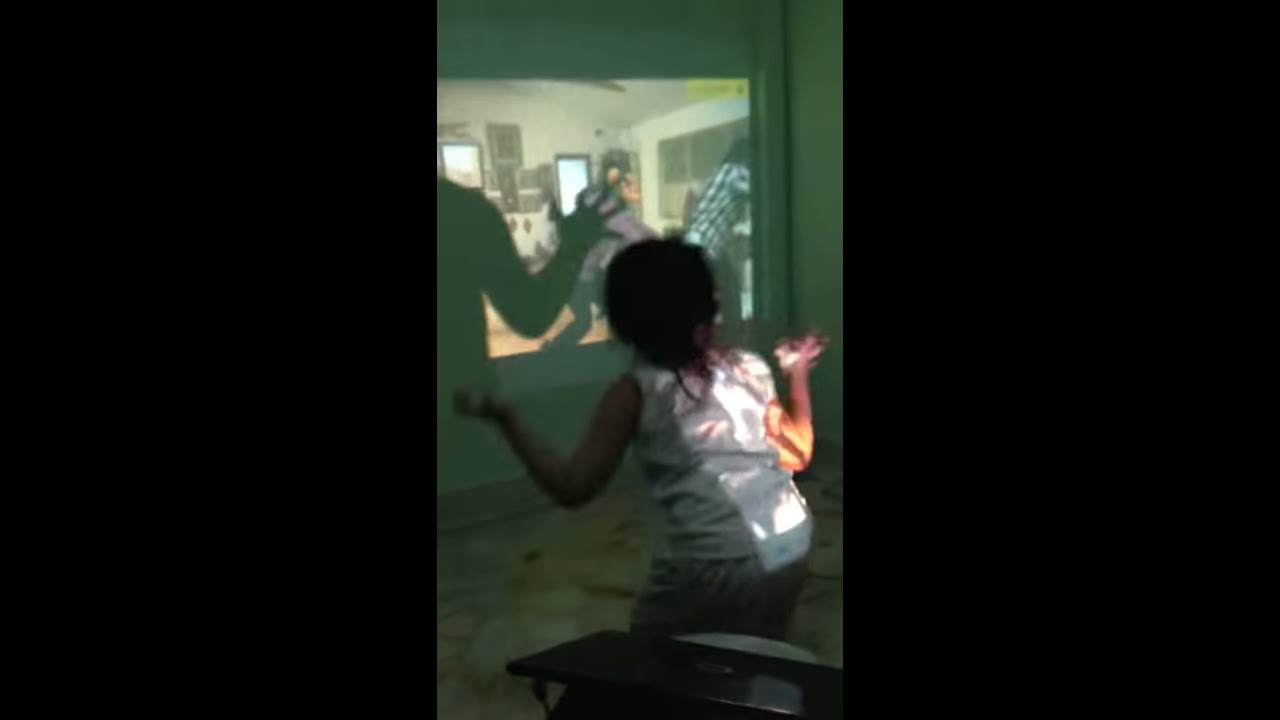The image showcases a young girl, approximately 6 to 10 years old, standing in front of a projector in what seems to be a dimly lit classroom or similar setting. The girl, with black hair possibly tied into a ponytail, is wearing a white short-sleeve shirt and grayish dark pants. She is standing with her elbows bent and her palms facing upward, creating an almost whimsical shadow on the whiteboard screen in front of her. The shadow, with her fingers spread out like monster claws, adds a playful element to the scene. Behind her, a black laptop rests on what appears to be a desk. The projected image on the screen seems to depict another room or classroom, featuring figures that include individuals in striped and purple shirts. The photo has vertical black borders on the left and right sides, framing the scene within a thin rectangular format. The overall image quality is grainy, making some details hard to discern, but the playful interaction between the girl and the projected image is clear and central to the visual narrative.